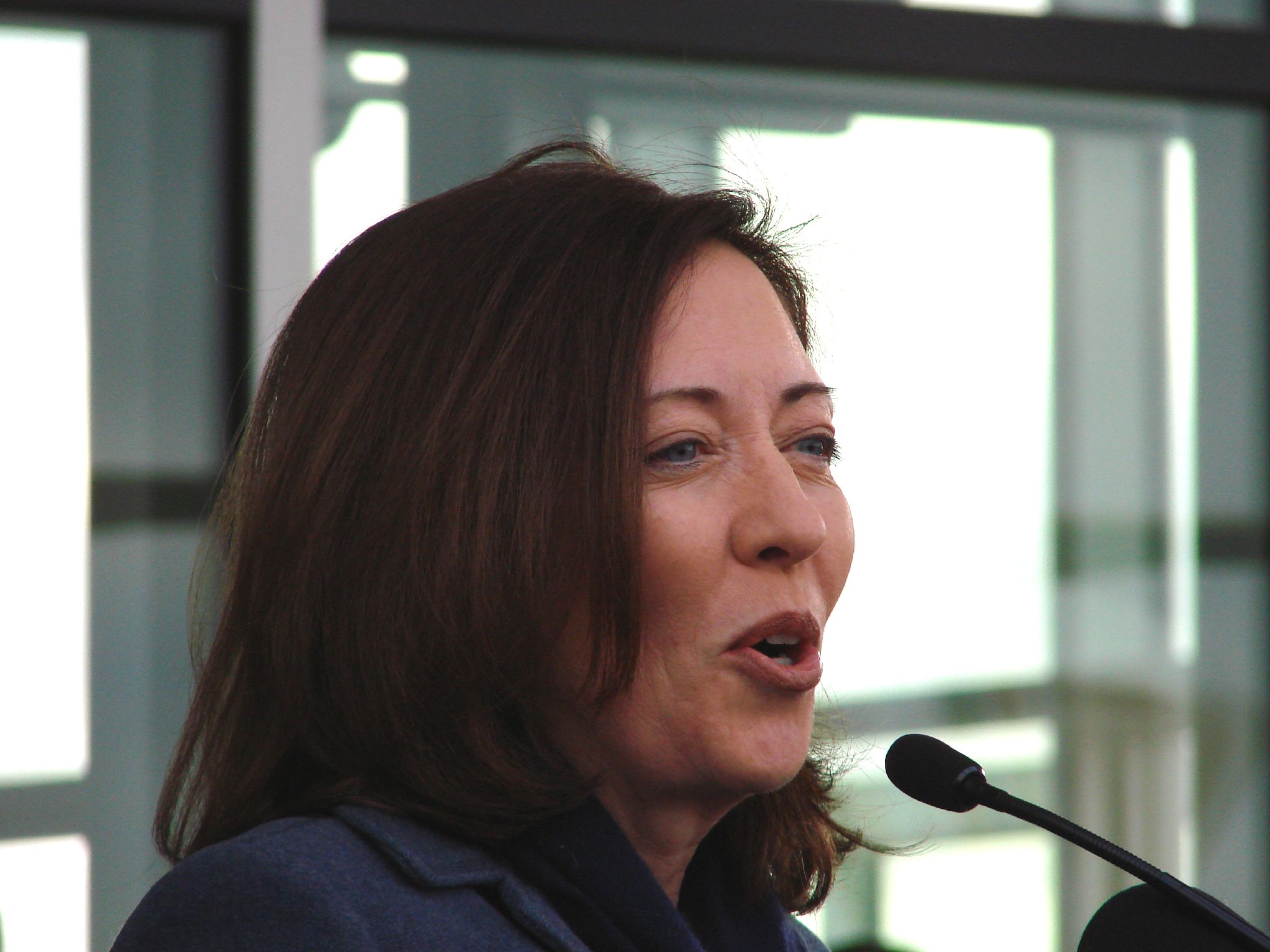This close-up photograph captures a woman with short brown hair and blue eyes, slightly turned to the right, speaking into a black microphone positioned on a podium. She is dressed in a dark blue coat, and her mouth is slightly open, as if she is mid-speech. The backdrop features an office setting with a window providing a soft white light, possibly due to cloudy weather or the reflection of a camera flash. The window, partially obscured by curtains on the sides, and additional window panes on the left merge into a blurred background, adding depth to the image while focusing on the woman's expressive face.